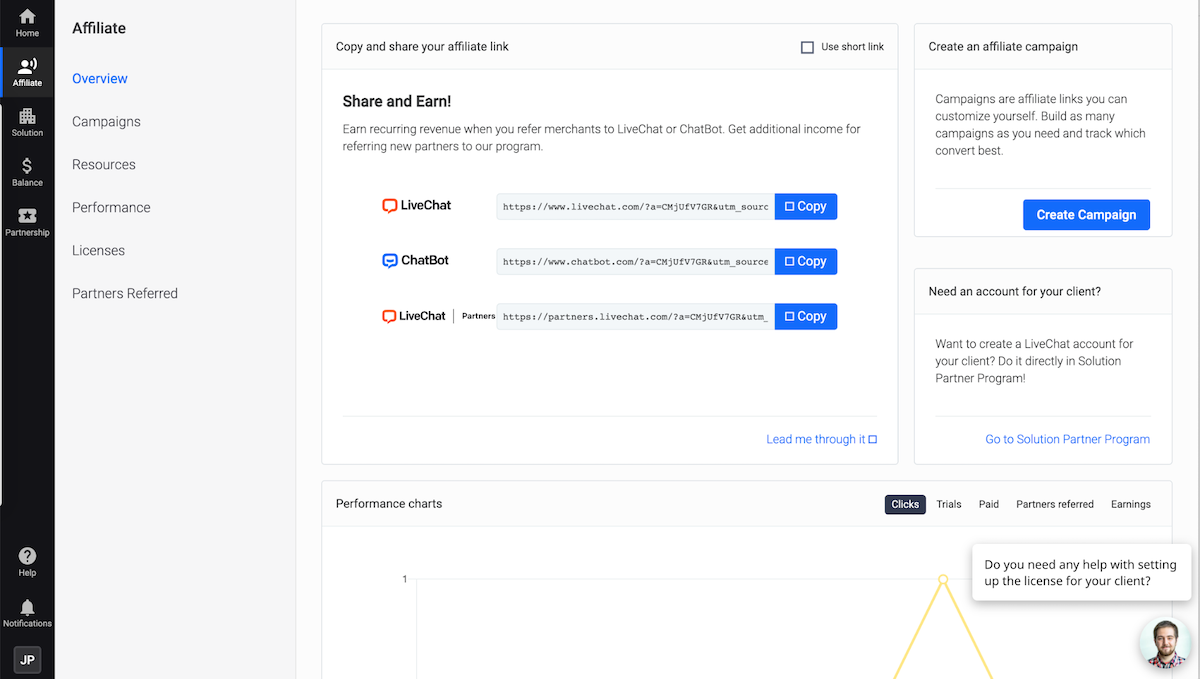This is a detailed screenshot from an unidentified website, illustrating various navigation menus and affiliate-related information. 

On the left side of the screenshot, a vertical menu is visible with options labeled "Home," "Affiliate" (which is currently selected), "Solution," "Balance," and "Partnership." Below these options are additional entries for "Help," "Notifications," and an entry labeled "JP."

To the right of this main menu, there's a sub-menu specific to the "Affiliate" section, featuring options such as "Overview," "Campaigns," "Resources," "Performance," "Licenses," and "Partners Referred."

The central section of the screenshot focuses on affiliate link management, prominently featuring a call-to-action to "Copy and Share Your Affiliate Link" along with an unselected option to "Use Short Link." The text encourages users to "Share and Earn," noting the potential for recurring revenue by referring merchants to LiveChat or Chatbot, as well as additional income for referring new partners. The affiliate links provided include:
- LiveChat, with a URL ending in "livechat.com/?A=CMJUFV7GR&utm_source"
- Chatbot, with a URL ending in "chatbot.com/?A=CMJUFV7GR&utm_source"
- LiveChat Partners, with a URL ending in "partners.livechat.com/?A=CMJUFV7GR&utm_source"

Each of these links has an associated "Copy" button which remains unchecked. Additionally, a checkbox labeled "Lead Me Through It" is visible, though it is not selected. 

The bottom part of this central section appears to discuss "Performance Charts," but the content is truncated and thus incomplete.

On the right side, the section elaborates on creating an affiliate campaign, indicating that users can customize links, build multiple campaigns, and track their effectiveness. Instructions to create a campaign and details about creating a LiveChat account for clients directly through the Solution Partner Program are provided, along with headings for tracking metrics such as "Clicks," "Trials," "Paid," "Partners Referred," and "Earnings."

In the bottom right corner, there is a photograph of a young, fair-skinned man with short hair and a dark beard. He is looking at the camera with a slight smile. A dialogue bubble above this image asks, "Do you need any help with setting up the license for your client?"

Overall, this screenshot offers a comprehensive view of the website's affiliate interface, including navigation menus, link management options, campaign creation guidelines, and support features.